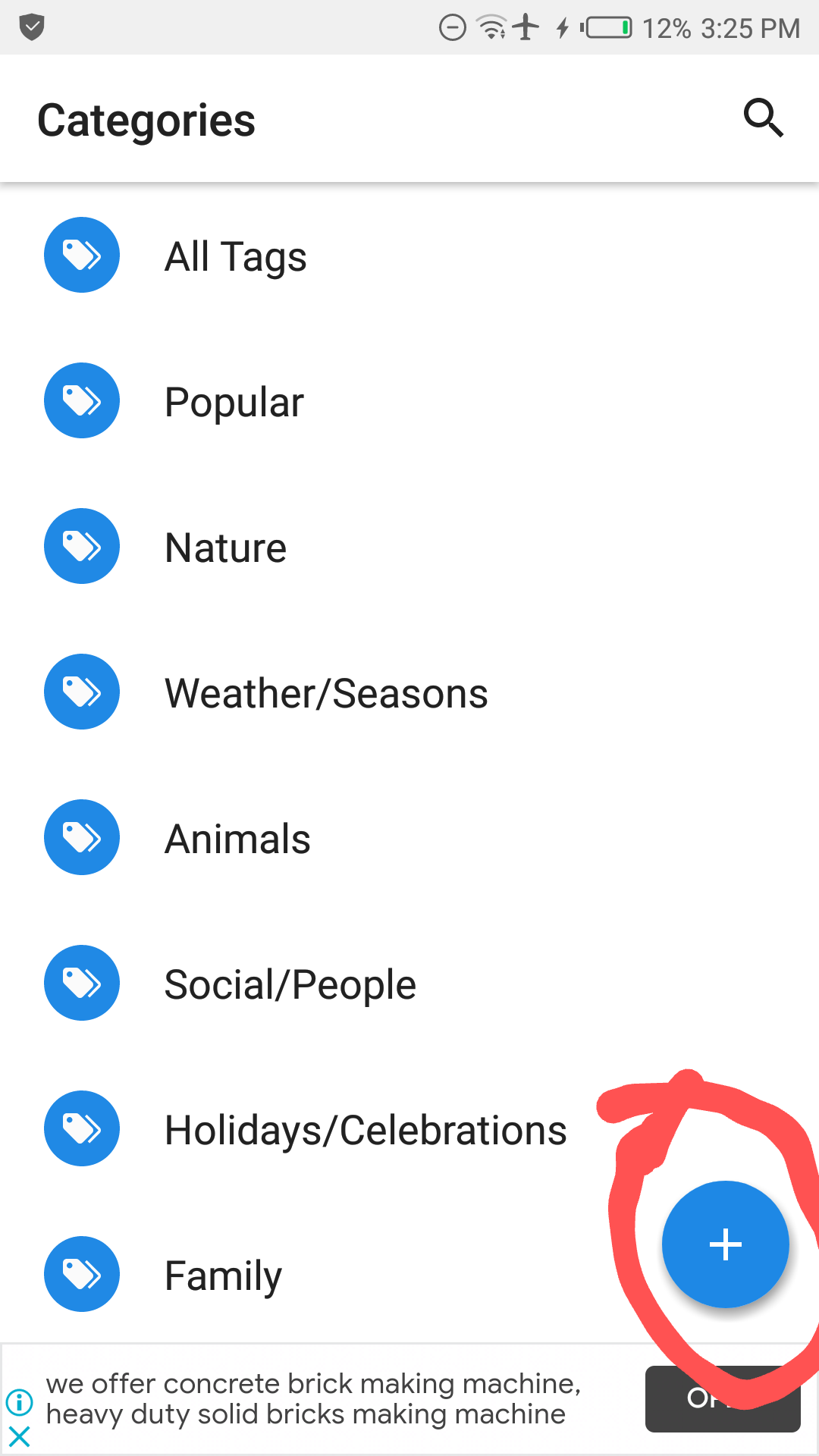The image appears to depict the screen of either a cell phone or a tablet. In the top left corner, there is an icon resembling a shield with a tick mark, likely indicative of an antivirus application such as McAfee. On the top right, there is an icon of a circle with a straight line through it, followed by a Wi-Fi symbol with an exclamation mark, suggesting connectivity issues. The Wi-Fi shows three bars, but the airplane mode is activated, aligning with the no internet access issue. The battery icon shows it is at 12% charge, and the current time is 3:25 PM.

Below the icons, the word "CATEGORIES" appears in black font on a white background. To the far right of this section is a magnifying glass icon, representing the search function. A grey line runs horizontally across the screen beneath these elements.

The section following the grey line features eight tags, each represented by a blue circle with a white tag icon inside. The tags are labeled in black text as follows: ALL TAGS, POPULAR, NATURE, WEATHER/SEASONS, ANIMALS, SOCIAL/PEOPLE, HOLIDAYS/CELEBRATIONS, and FAMILY. Set prominently next to these tags is a blue circle with a white plus sign inside, encircled by a bold hand-drawn outline, indicating it is used to add new tags.

At the very bottom of the screen, there is an advertisement stating: "WE OFFER CONCRETE BRICK MAKING MACHINE. HEAVY DUTY SOLID BRICKS MAKING MACHINE."